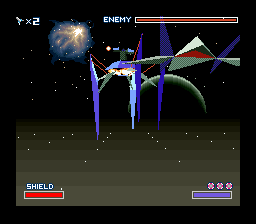This screenshot is from the classic Super Nintendo game, Star Fox. Recognized as one of the pioneering titles on the console, Star Fox utilized the innovative Super FX chip, which enabled it to render impressive 3D graphics for its time. In this particular image, we see the player's spacecraft engaging in combat, as indicated by the laser blasts aimed at an enemy boss. The enemy's health bar is prominently displayed, adding to the intensity of the battle scene. This game remains a standout example of early 3D gaming on the Super Nintendo.